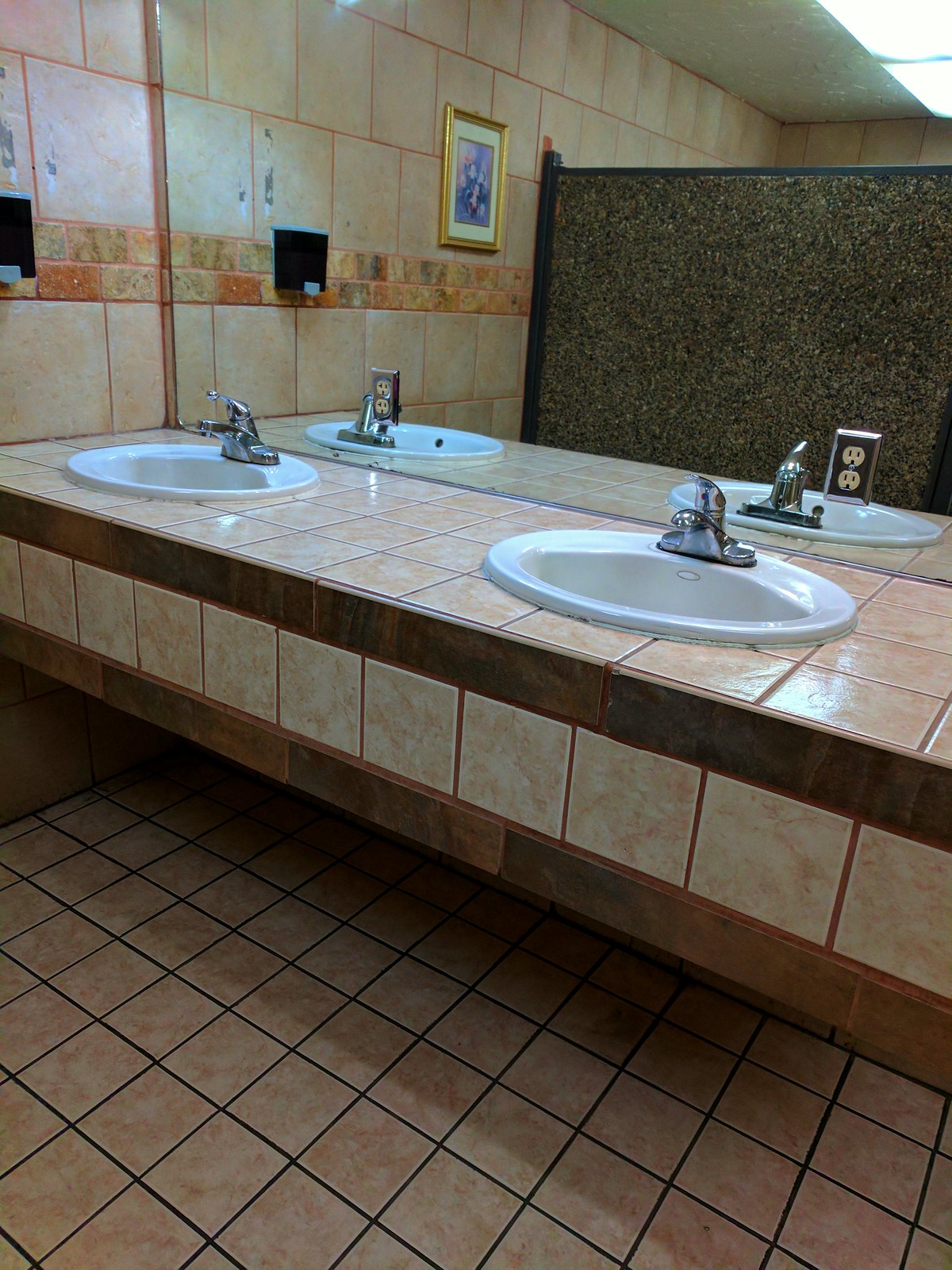The image captures a well-lit, commercial or restaurant restroom featuring an elegant sink area set in a tan marble-style countertop. The counter has lighter brown tiles with a darker brown outline and is supported by dark-stained wooden boards. Prominently, two white ceramic sinks with single-lever silver faucets are positioned side by side. Adjacent to and behind each sink, there is a power outlet, which, along with the sinks, is reflected in a large mirror mounted behind them. Visible in the reflection are a wall of stall doors with a dark brown and white speckled material, a soap dispenser, and a framed photograph on the back wall. The shot angle also highlights the clear and well-defined lighting provided by the overhead fluorescent lights.